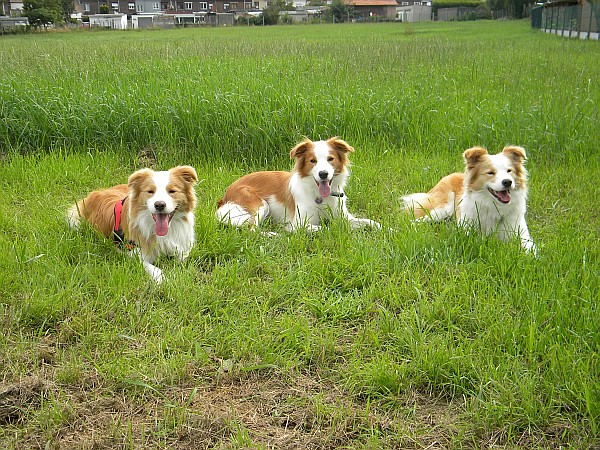In this detailed image, we see three nearly identical collies lounging on a lush, very green grassy field on what appears to be a hot day, as all three dogs are panting with their mouths open and tongues visible. Each collie boasts a striking pattern of thick white and light brown fur: their chests and the middle portions of their faces are adorned with white fur, while the cheeks, ears, backs, and haunches are cloaked in brown. One collie wears a red harness, another sports just a collar, and the third has no neck apparel. The dogs are intently staring towards the camera, creating a captivating sense of engagement.

In the background, a fence runs along the upper right-hand side of the image, potentially marking the boundary between two fields. Behind this, tall grass can be seen leading up to a small town in the distance. The town features dark brown and gray buildings, with visible windows, which might be houses or apartment complexes. The scene exudes a rustic, pastoral charm, framed by the serene presence of the collies.